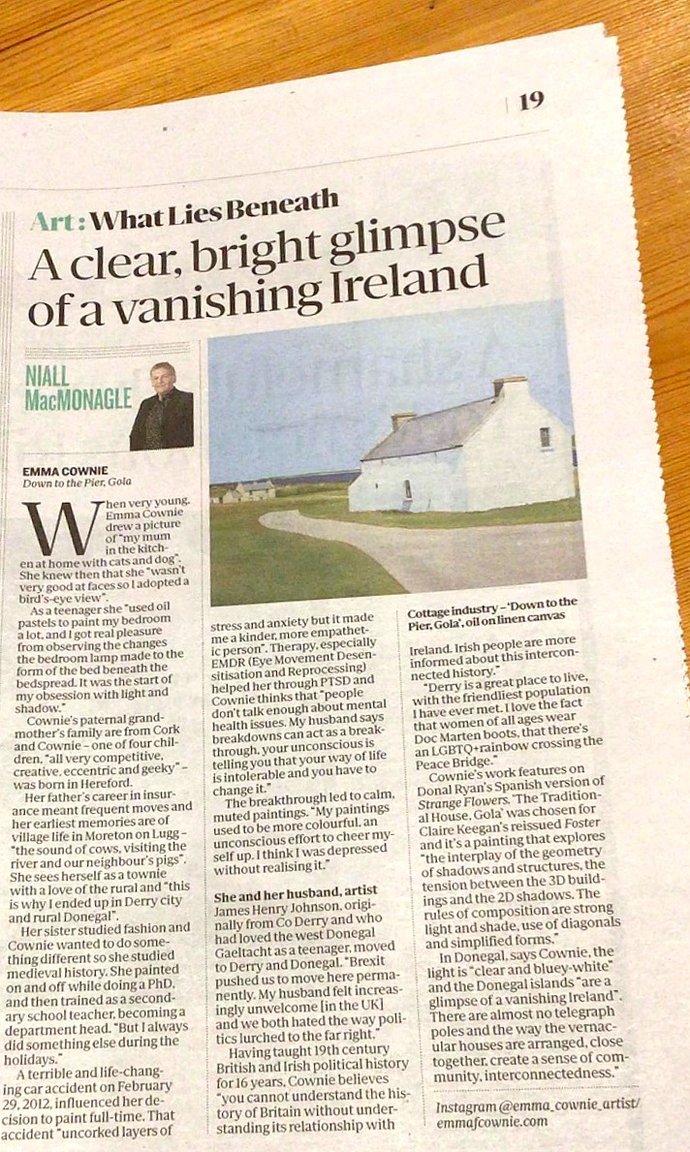A detailed caption for the image described:

---

Title: "What Lies Beneath? A Clear Glimpse of a Vanishing Ireland by Niall McMahon"

This screenshot captures page nine of a newspaper's art section, featuring the article "What Lies Beneath? A Clear Glimpse of a Vanishing Ireland" by Niall McMahon, with contributions from Emma Crown. The article is divided into three sections and showcases an evocative image: a winding path leading through a countryside scene with quaint houses on either side. Niall McMahon, dressed in a suit, oversees this picturesque exploration of rural Ireland. The jagged edges of the newspaper hint at a hands-on approach to its presentation. The page rests on a wooden table with a grainy yet natural finish, adding to the rustic charm of the setting. For more about this project and the artists involved, visit Instagram @EmmaCountyArtist, where you can explore the quaint cottage industry down to the pier.

---